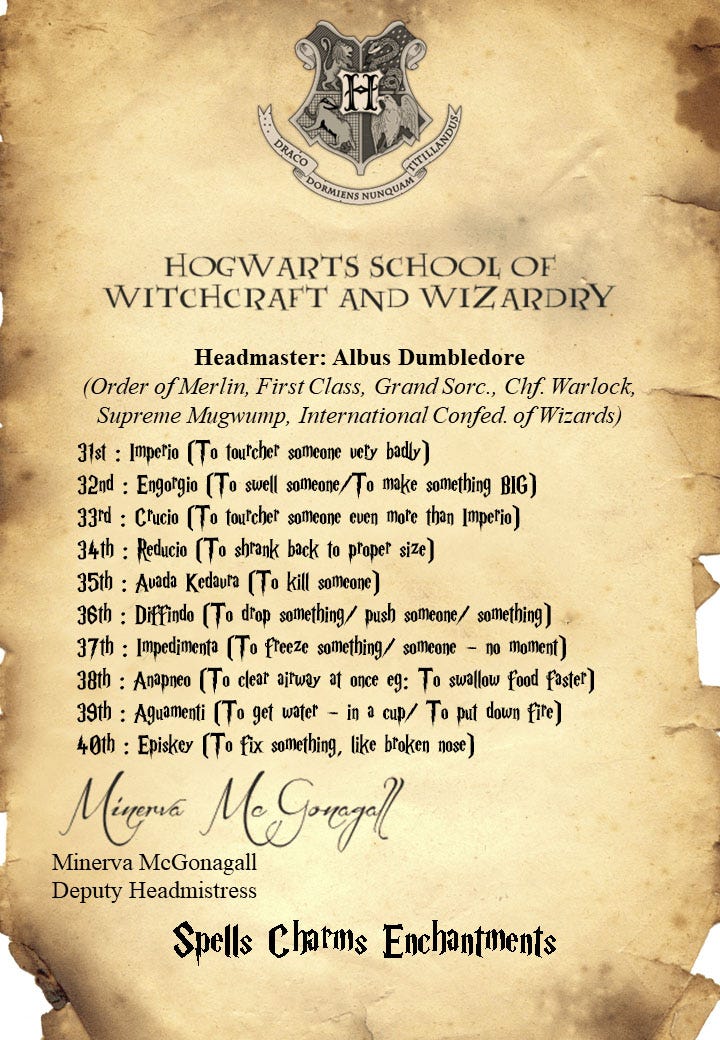The image depicts a simulated piece of old-school parchment paper, weathered and torn as if lifted straight out of the Harry Potter universe. At the top, the parchment prominently features the Hogwarts School of Witchcraft and Wizardry crest, showcasing the lion, snake, badger, and eagle. Below the crest, a banner reads “Draco Dormiens Nunquam Titillandus.” 

The header includes the text "Hogwarts School of Witchcraft and Wizardry" rendered in the iconic Harry Potter font. Beneath this, the parchment lists Headmaster Albus Dumbledore's extensive titles: Order of Merlin, First Class, Grand Sorcerer, Chief Warlock, Supreme Mugwump, and International Confederacy of Wizards.

Following Dumbledore's titles, the parchment documents a series of spells and their effects, numbered from the 31st through the 40th. These spells include:

- 31st Imperio: to control someone completely.
- 32nd Engorgio: to make someone or something swell.
- 33rd Crucio: to inflict immense pain.
- 34th Reducio: to shrink someone or something back to proper size.
- 35th Avada Kedavra: to kill someone.
- 36th Defendo: to repulse or fend off something or someone.
- 37th Impedimenta: to freeze or obstruct movement.
- 38th Anapneo: to clear someone's airway.
- 39th Aguamenti: to conjure water or extinguish fire.
- 40th Episkey: to heal minor injuries.

The parchment is signed by Minerva McGonagall, identified as the Deputy Headmistress in charge of Spells, Charms, and Enchantments. The detailed and rich styling of the document, with its calligraphic text and traditional design elements, evokes a sense of authenticity as if it were an artifact directly from the Harry Potter films.